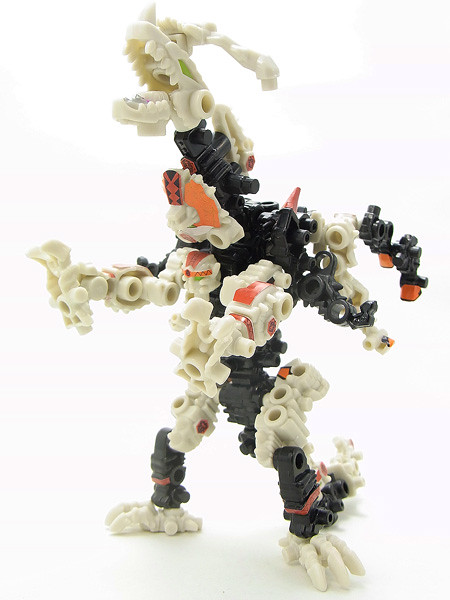The image depicts a large, plastic toy resembling a robotic dragon or dinosaur, meticulously constructed using snap-together pieces akin to Legos or K'nex. Predominantly black in color, this intricate model features white elements on its head, paws, and armor, along with accents of orange and possibly a touch of yellow. The toy, composed of approximately 30 to 50 individual parts, stands upright on its back legs with its jaw wide open in a roaring pose. Notably detailed, it includes potential wings extending from its back, adding to its imposing and dynamic appearance. The backdrop and the floor in the image are both white, emphasizing the toy's bold color contrasts.